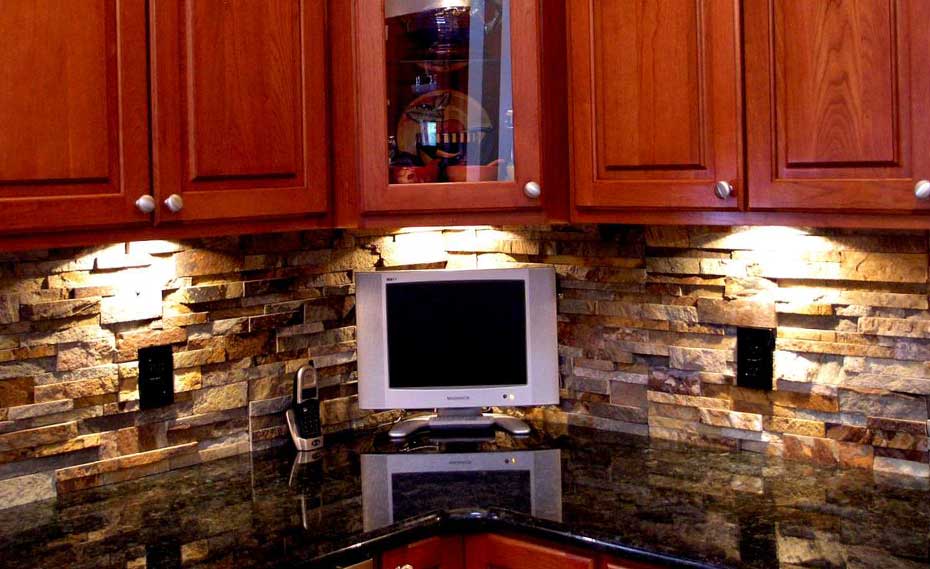The photograph captures a portion of a rustic kitchen with a distinct, textured stone wall made up of variously sized bricks. The upper part of the image showcases five dark wood cabinets; each adorned with unique cutouts, and arranged in a pattern with two on the left, a single central cabinet with a clear glass door, and two more on the right. The glass-fronted central cabinet reveals a collection of colorful dishes inside. There are lights installed under each pair of cabinets, illuminating the scene and casting reflections on the gleaming, black countertop below.

Underneath the cabinets, three light switches are visible along the brick wall. The countertop, highly polished and shiny, mirrors the surrounding elements, including the computer monitor stationed centrally below the middle cabinet. Just to the left of this monitor appears to be a cell phone, although some reflections on the glossy surface may create visual confusion. The counter extends to form a 90-degree angle, further accentuating the rustic and modern blend of the kitchen space.